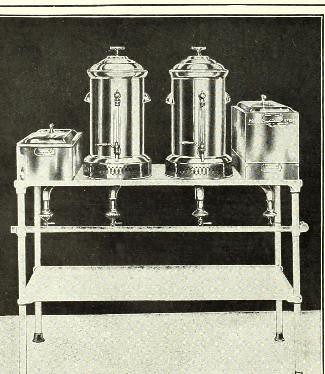The black and white image depicts a stationary metal cart, likely designed for storing and dispensing hot food or beverages. The cart features two distinct levels: a bottom layer which is empty, and a top layer that holds two cylindrically shaped steel silos and two steel boxes. The layout on the top layer is organized with a box on one end, followed by a silo, another silo, and another box.

Each of these containers, both the silos and the boxes, is equipped with a metal faucet or valve at the bottom, indicating their function as dispensers. The cylindrical silos are positioned centrally, while the boxes are situated on either end of the top layer, with the left box being smaller than the one on the right. The overall finish of the cart and its containers suggests an old or vintage nature, adding to the monochromatic aesthetic of the photocopy.

The cart itself has four steel legs and lacks wheels, making it stationary. The depiction of shadows and highlights, especially the shine on the metallic surfaces, emphasizes the reflective quality of the steel. The entire setup, from the metal structure to the containers and pipes, is rendered in shades of grey, giving the image a stark and industrial feel.